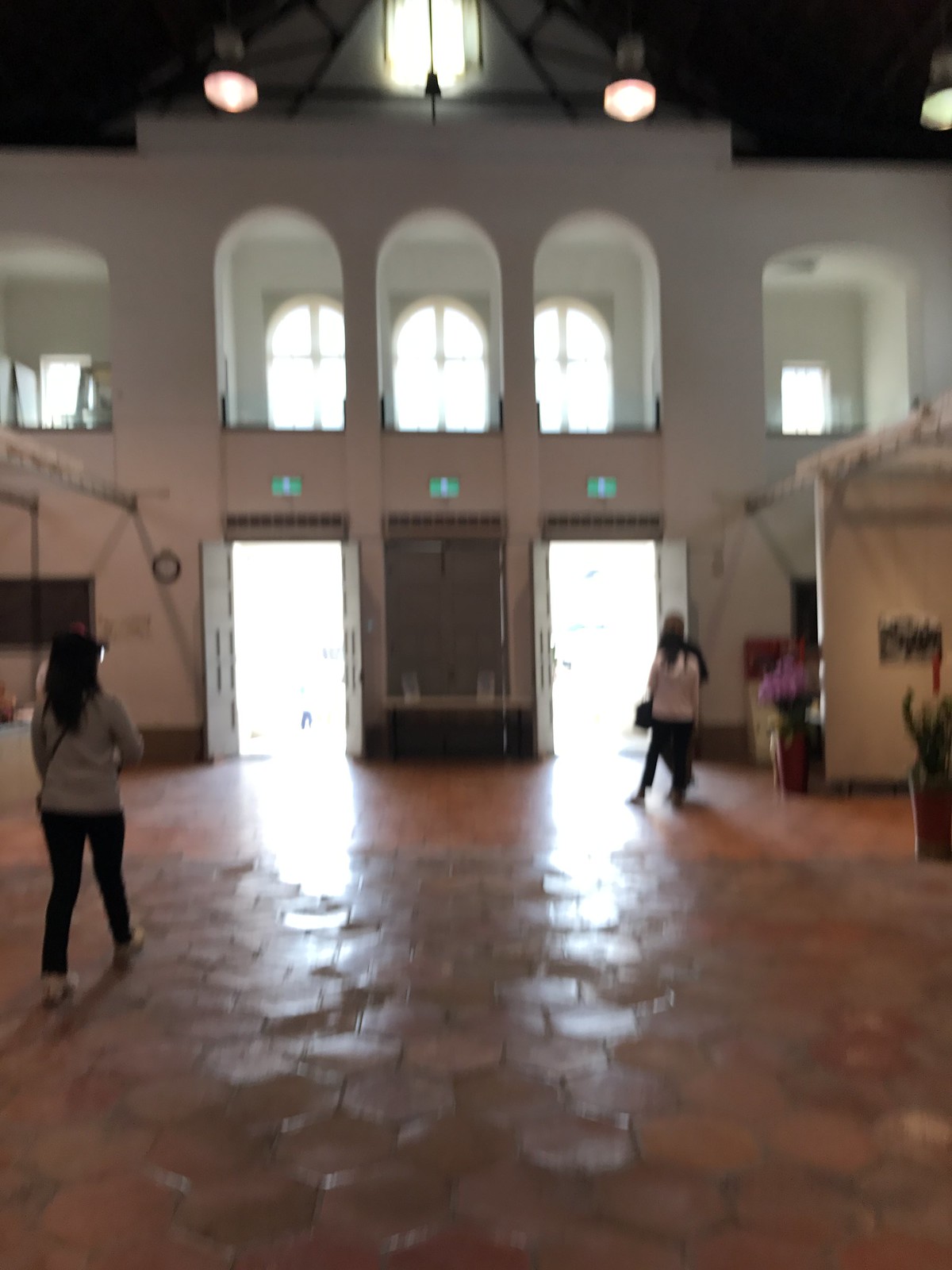The photograph captures an expansive, indoor space with an air of grandeur, indicative of a commercial building, museum, or church. The flooring is distinctive with red hexagon-shaped tiles that cover the ground extensively. Unusually high ceilings feature arched windows that allow natural light to flood the area. Several people are seen walking within the space; notably, a woman on the left side is dressed in a light-colored shirt and dark pants, her long dark hair adding to her recognizability. Towards the center-right of the image, two other individuals are seen, although their features are blurred and out of focus. Around the edges of the room are potted plants and flowers, adding a touch of nature to the otherwise architecturally focused setting. The photograph is free of any text, allowing the visual elements to speak for themselves.